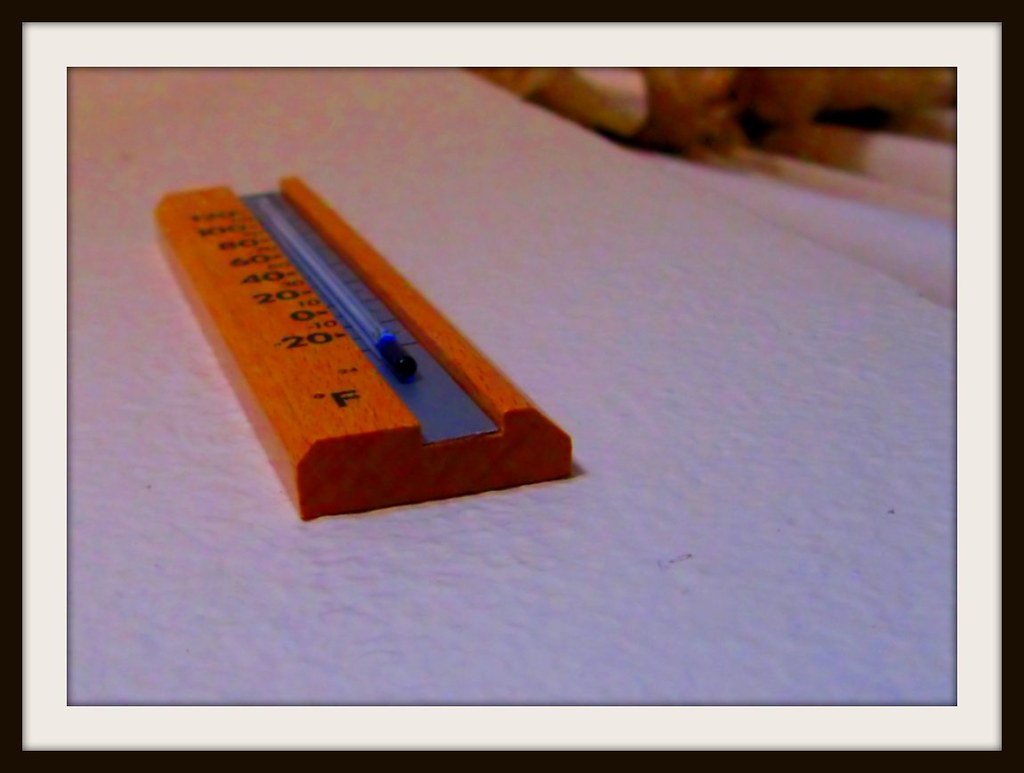The image captures a wooden Fahrenheit thermometer resting on a textured surface, which might be a blanket due to the visible wave in the upper right-hand corner. The thermometer, framed with a white matting and enclosed by a black border, features etched black measurements along its left side. The glass tube at the center of the wooden frame lies against a black middle section. In the background, indistinguishable objects, possibly stuffed animals, cast faint shadows. A hint of blue substance is seen at the bottom of the thermometer, though the exact temperature reading itself is not visible.